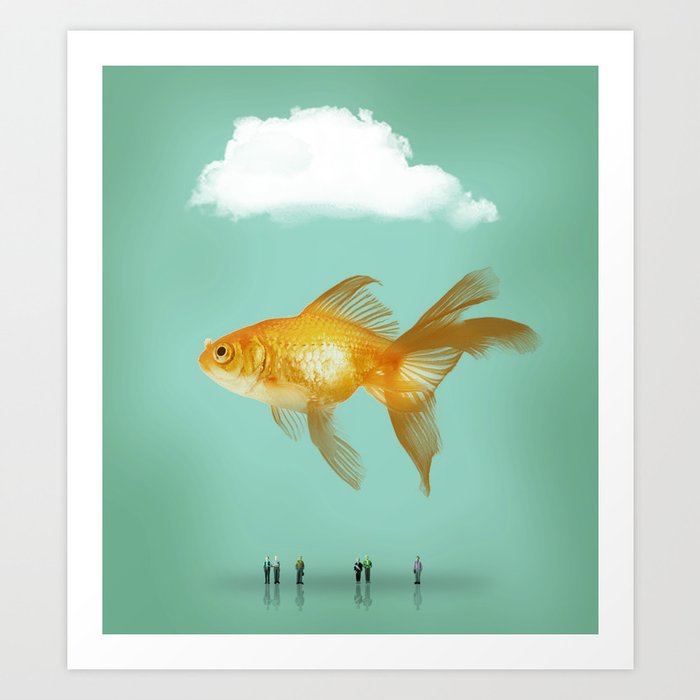This image is a meticulously crafted piece of artwork featuring a central, oversized, and highly realistic goldfish, seemingly floating beneath a large, puffy white cloud. The backdrop is a blue-green gradient, creating a serene and surreal atmosphere that doesn’t resemble water but rather an artistically chosen background color. Below the goldfish are six diminutive individuals, whose details and attire are largely indistinct, save for one in a green shirt and another in purple, both appearing to have white skin. Their shadows are faintly reflected, suggesting the presence of a reflective surface, possibly water or glass, though only the middle two appear to be interacting directly with it. The composition hints that these tiny figures are standing on a sandy or murky surface, gazing up at the goldfish as if in awe. The dramatic scale between the giant goldfish and the minuscule people gives a surreal and almost whimsical quality to the image. The entire scene is enclosed within a minimalist white frame, adding a polished touch to the artwork, which appears to be displayed on a white wall.